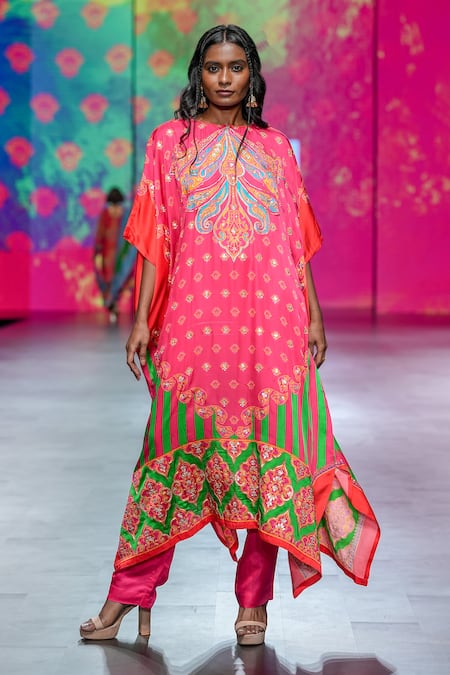The image features a South Asian woman with deep brown skin and long, curly black hair, parted in the middle and adorned with braids framing her face. She is standing confidently against a vibrant, tie-dye backdrop of hot pink and blues, suggesting a runway show. The runway appears to have a cement floor. The woman is dressed in a colorful and intricate South Asian outfit, consisting of hot pink pants and a flowy tunic. The tunic is predominantly pink with a gradual transition of patterns and colors, featuring a large emblem in the middle adorned with turquoise, purple, and yellow hues. The lower part of the tunic has a mix of green and pink with detailed patterns, ending in a drapey, handkerchief hem. She accessorizes with large gold earrings and natural leather tan heels with a strap over her toes. Her nails are unpainted, and she wears makeup, enhancing her elegant and poised look as she models the attire.